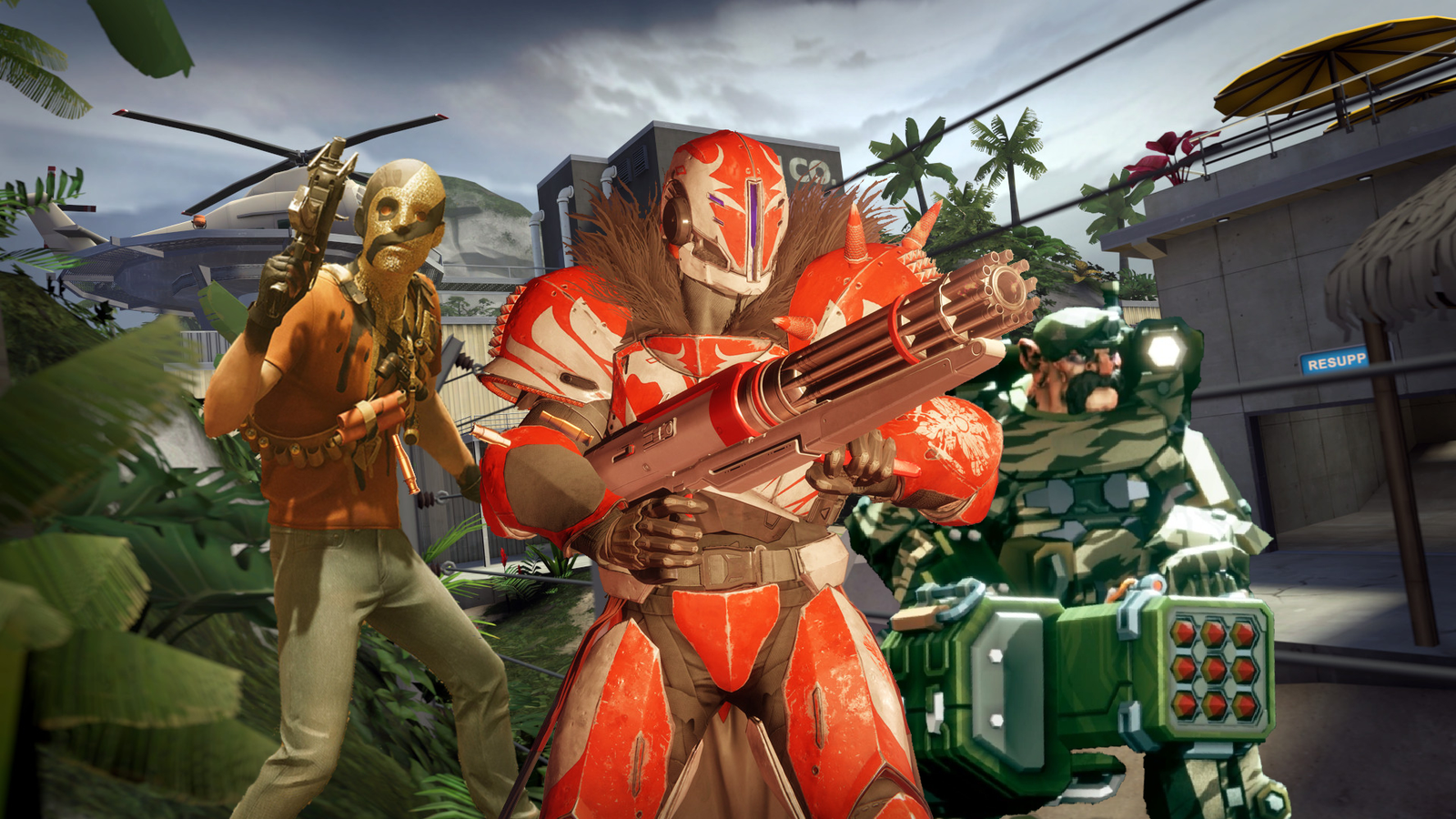The image depicts a vibrant and action-packed scene featuring several diverse characters and a detailed background. Central to the image is a hero clad in a red armored suit, reminiscent of a Power Ranger, who is wielding a large copper-colored machine gun adorned with red rings. His helmet, with red and off-white hues, covers his face and has soft, almost feather-like details on the sides. The figure is adorned with protective gear, including a brown belt and leg, groin, and shoulder armor, all richly detailed.

To the right of this central figure, a man in camo attire is seen. He sports a large mustache and wears a green camo helmet. He seems to be riding in some sort of vehicle and is holding a piece of machinery, possibly a machine gun or bomb launcher. This character is also depicted with a green outfit, blending seamlessly with his surroundings.

On the far right, there is a gray building with the word "RESUP" displayed in white letters against a bright blue background. Atop this building is an umbrella typically found on outdoor tables. Further enhancing the scene are palm trees, other foliage, and a somewhat bright, though progressively darker toward the left, sky.

On the left side of the image stands another character, this time wearing brown pants and an orange shirt. This individual is bald and has a gold protective covering on his face. He holds a futuristic weapon, not a traditional gun but something potentially dangerous. There is also a helicopter in the backdrop, colored gray with hints of blue, and surrounded by leaves and ferns.

Together, these elements create an intense, action-oriented tableau, packed with dramatic details and vivid elements.